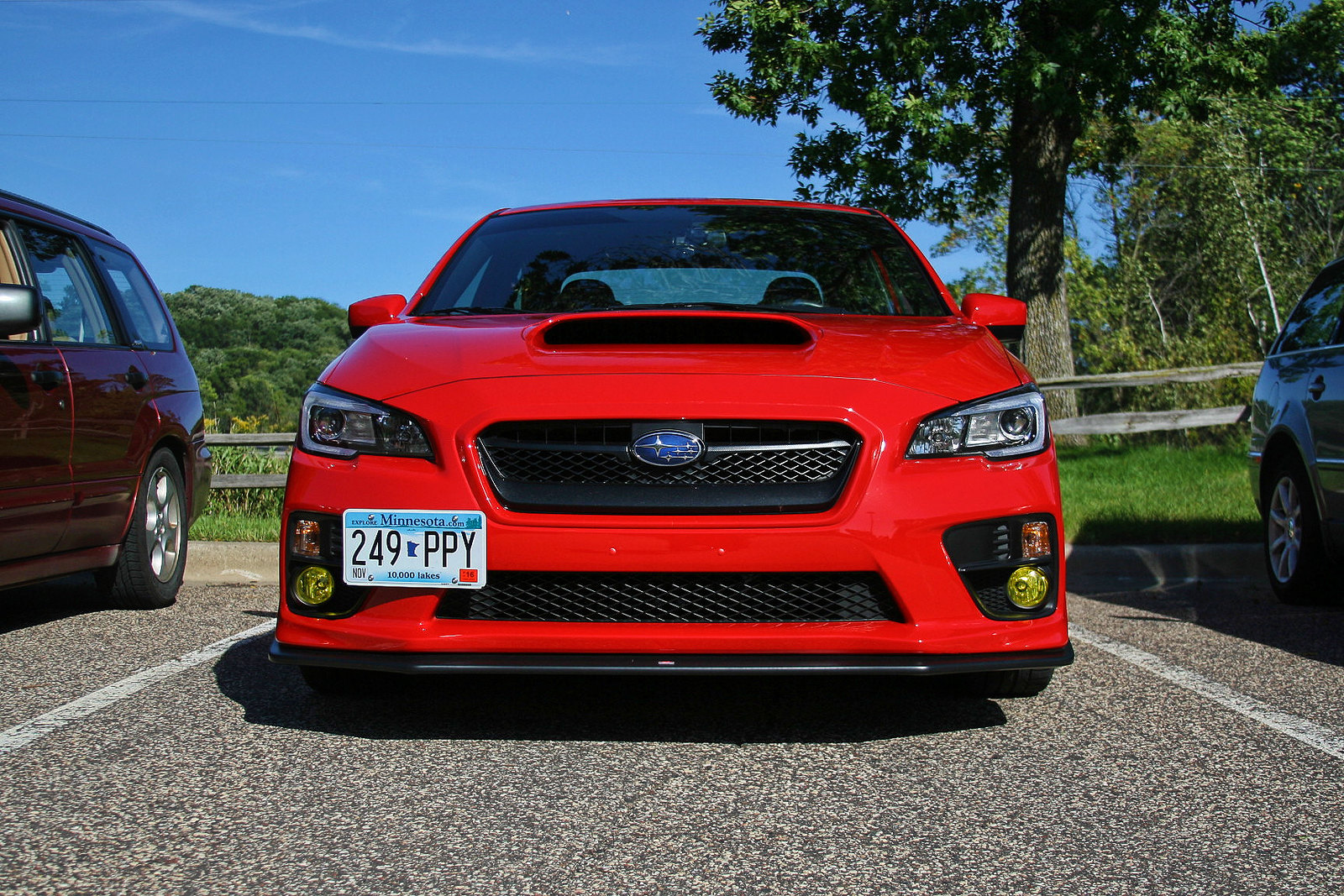This photograph, taken outdoors during the day, captures the front view of a red Subaru perfectly parked in a designated spot within a paved parking lot with distinct white lines demarcating the spaces. The focal point, this Subaru, boasts clear headlights and small yellow circular fog lights at the bottom, with amber blinkers positioned beside the headlights. Its hood features a noticeable vent, and prominently displayed on the grille is the iconic blue Subaru logo adorned with four silver stars. The Minnesota license plate, numbered 249PPY, is affixed to the lower left-hand side of the front bumper. Flanked by two vehicles, the rust-colored station wagon to the left and a dark green four-door sedan to the right, the red Subaru stands out. Beyond the pavement, there is green grass, a wooden fence, and a tree on the right-hand side, all under a clear blue sky, indicating a pleasant and likely warm day.